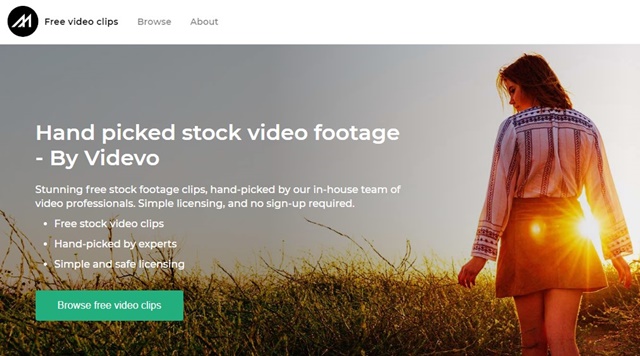The web page features a clean, white header bar. On the left side of the header, there is a black circle icon with a white "M" inside it, followed by the text "Free Video Clips." To the right of this icon, options for "Browse" and "About" are displayed. The main content of the page is dominated by a photograph with superimposed text. The photograph shows a gray, overcast sky in the background and a meadow-like landscape in the foreground. On the right side of the image, a woman can be seen wearing a striped blouse and a short orange skirt, with bright sunlight filtering through the space between her skirt and arm. The overlaid text reads: "Handpicked Stock Video Footage by Videvo. Stunning free stock footage clips handpicked by our in-house team of video professionals. Simple licensing. No sign up required. Free stock video clips handpicked by experts. Simple and safe licensing." Below this text, a prominent green button invites users to "Browse the free video clips."